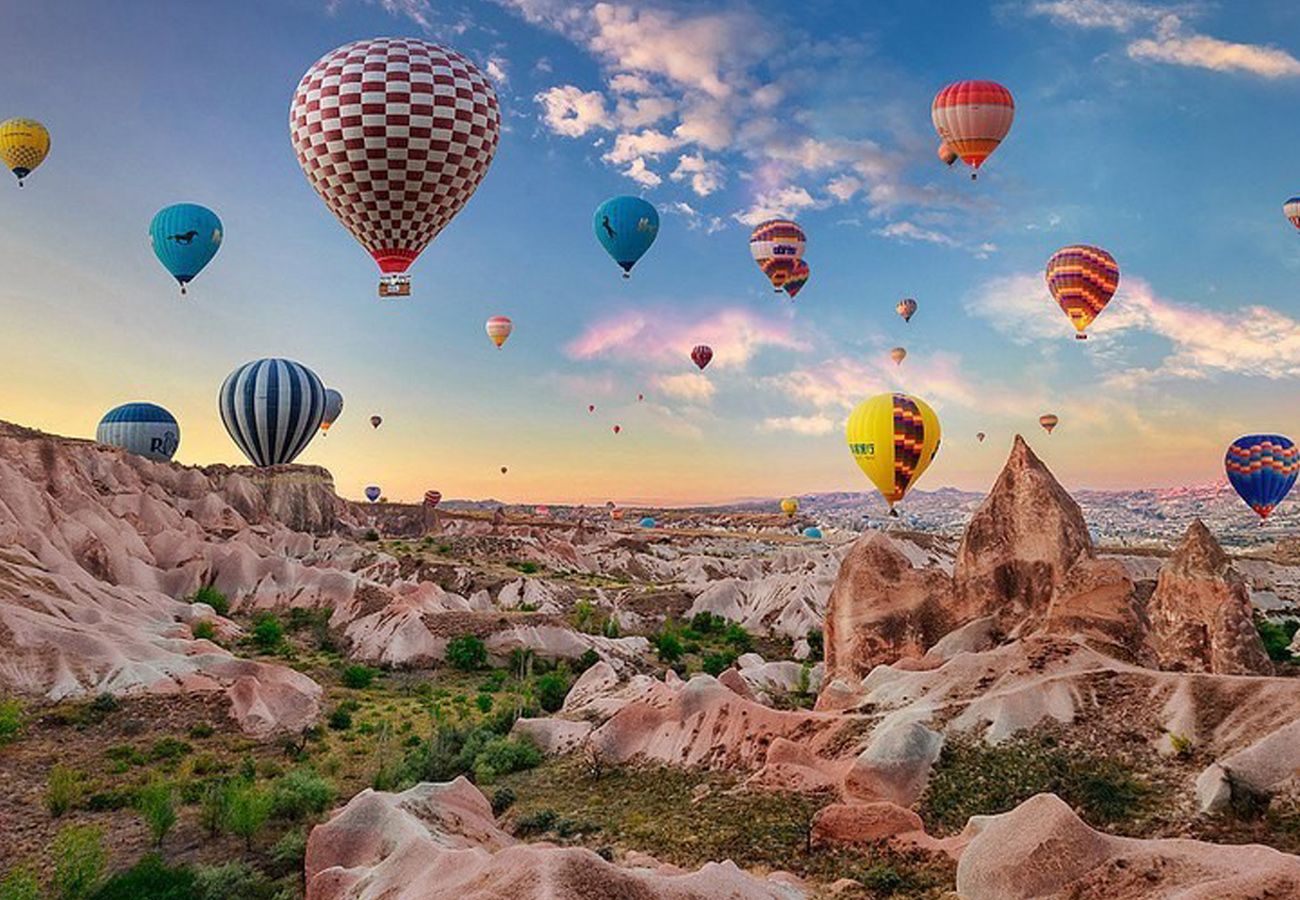This outdoor photograph captures a breathtaking scene of dozens upon dozens of hot air balloons soaring in the sky at dawn or dusk. The sky transitions from a deep blue above to a vibrant orange-yellow near the horizon, indicating the early morning or late afternoon light. Scattered white clouds add texture to the sky.

In the center-left of the image, a red and white checker-patterned balloon stands out, while to its left, a blue balloon with a black horse running across its side adds a whimsical touch. The balloons, which number perhaps over a hundred, float serenely above a rugged, rocky landscape.

The foreground features red, rocky ridges and small cliffs interspersed with green shrubs and grasses. Towards the right, three notably sharp rock formations jut dramatically into the sky, although the balloons remain well above these natural spires. In the distance, more balloons are visible, hovering over similar rocky outcrops and a small village. The backdrop is completed by distant gray mountains, enhancing the majestic ambiance of this vibrant, scenic view.